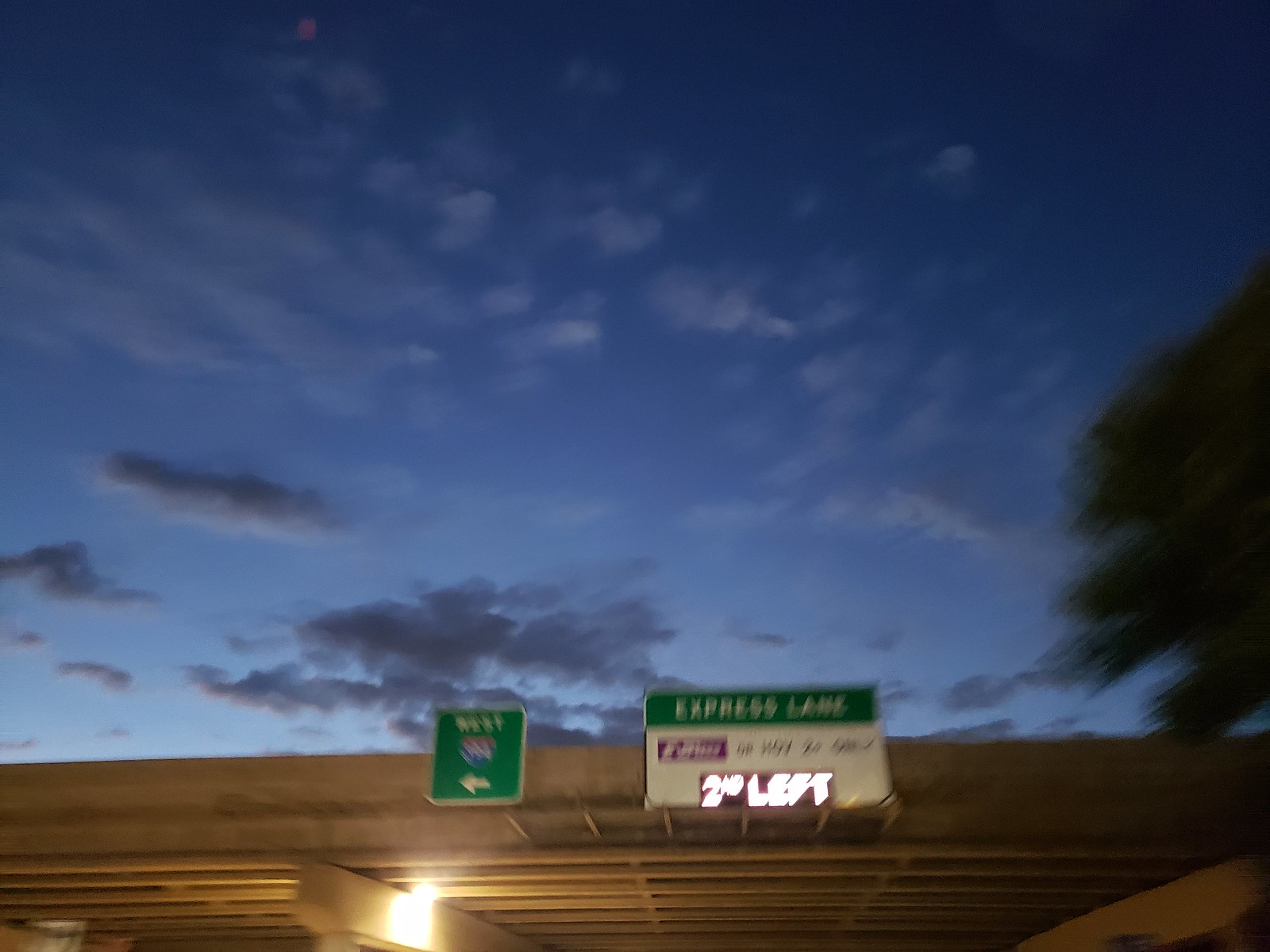The image depicts a blurry photograph captured from a moving vehicle, showcasing an overpass or bridge enveloped in a dark setting. The photograph is noticeably unclear, making the text on the road signs difficult to read. Some parts of the blue sky, punctuated with shadowy clouds, are visible in the background. A blurred silhouette of a tree can be seen in the frame, adding an element of nature to the urban scene. The roadway leads towards the bridge or overpass, indicating imminent passage under it. Prominently displayed are two road signs: a square green sign with the word "West" and an arrow pointing to the left, and a rectangular sign bearing the phrases "Express Lane" and "Second Left."